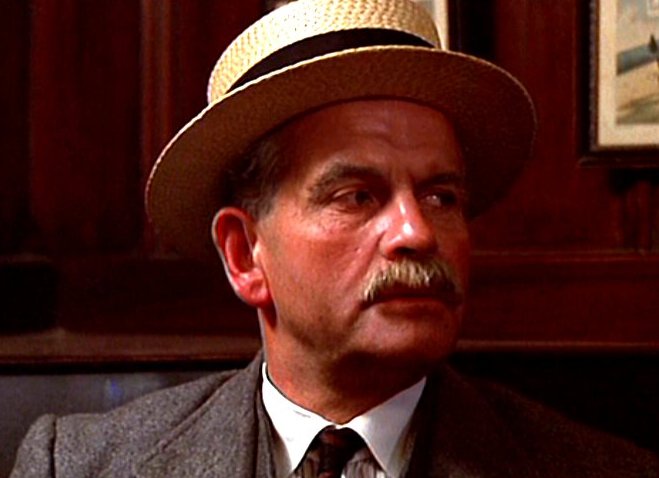The image features a detailed portrait of an elderly man, appearing to be in his late 50s or early 60s. He is a white male, clean-shaven, with a distinguishable grayish-blonde mustache. His skin is noticeably red and marked with pock marks, and his hat, a textured tan piece that has a black band around the middle resembling straw or wicker, covers most of his hair, although some gray is visible at the sides. The gentleman gazes to his left. He is dressed in a gray wool-type suit with a matching vest, a white shirt, and a burgundy-black collar, possibly a tie. The background reveals a wooden wall adorned with framed photos, one of which is partially visible in the top right corner, featuring a white border.